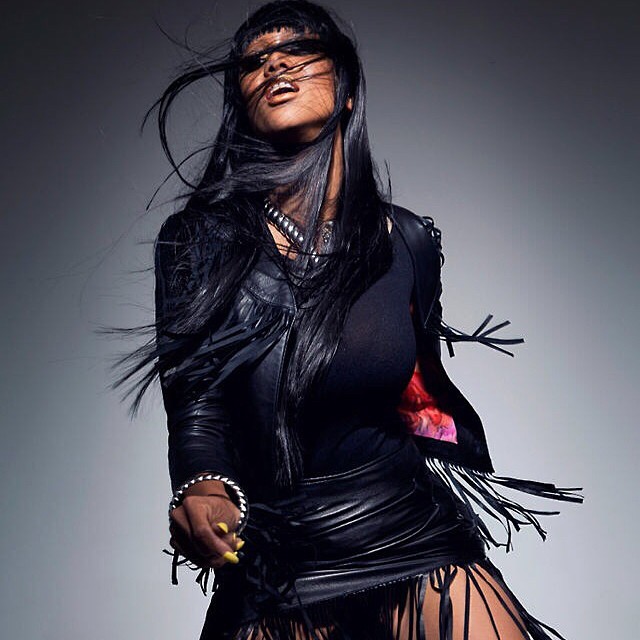The photograph resembles a fashion magazine spread, featuring an African-American woman with strikingly long, straight, glossy black hair that is being whimsically blown around, giving the image a dynamic sense of movement. Her short, straight-cut bangs create a sharp, stylish contrast against her flowing locks, some of which partially obscure her eyes. The background transitions from a light gray at the bottom to a darker gray or blue-purple at the top, adding depth and highlighting her presence in the center of the frame.

She is dressed in a dark purple, long-sleeved leather jacket with fringes, which complements her matching dark attire. The fringes of her short leather skirt echo the lively motion of her hair. She accessorizes with a chunky silver necklace and a silver bangle bracelet on her right wrist, while her fingernails are painted a distinctive yellow.

The overall scene is artistically captured, with her mouth slightly open revealing her top teeth, and her chin elevated, suggesting confidence and poise. Strands of her hair are blown across her face and eyes, and around her neck, adding to the sense of fluidity and movement in this captivating, high-fashion photograph.